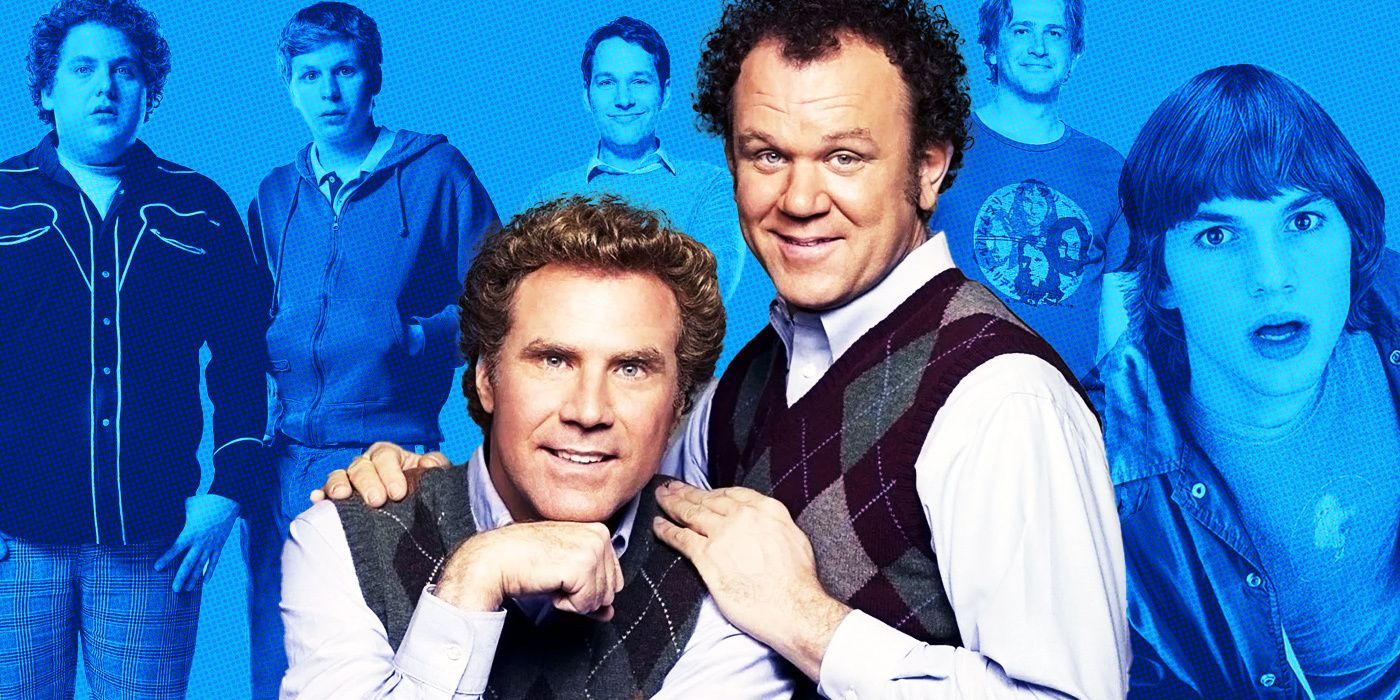The composite image features a collection of prominent comedic actors and the characters they portray. Dominating the foreground in vibrant color are Will Ferrell and John C. Reilly, posing as their characters from the movie "Step Brothers." They are dressed in contrasting sweater vests and lavender button-down shirts, exuding a professional family portrait vibe as they smile directly at the camera. In the background, the image transitions to a light blue shade, showcasing additional actors in a more subtle tone. From left to right, we see Jonah Hill and Michael Cera from "Superbad," followed by Paul Rudd, known for his role in "Ant-Man." An unidentified actor wearing a t-shirt with a possible Beatles design stands next, and to the far right is Ashton Kutcher. The overall setting is bright and well-lit, clearly highlighting the distinct color contrast and detailing in the actors' attire and expressions.